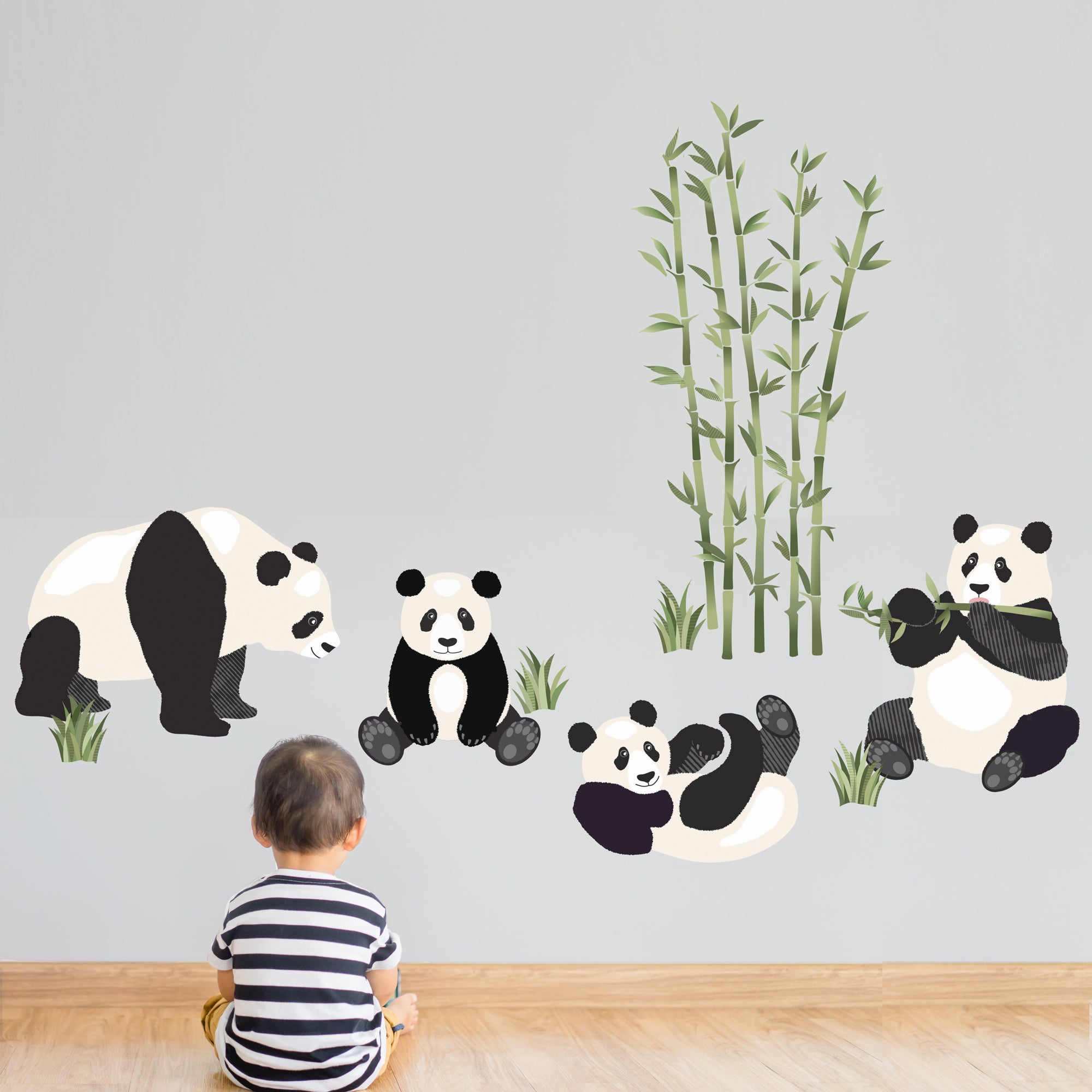In this image, a young child, approximately 3 or 4 years old with short, dark black hair, is seated on a light brown hardwood floor, facing a gray wall adorned with illustrations of panda bears. The child is positioned in the bottom left of the picture, and we see the back of his head as he intently observes the artwork. He is wearing a black and white striped shirt, with his arms held in front of him. On the wall, there are four distinct panda bears:

1. On the far left, a panda bear stands on all four legs, which are notably longer in the front, giving it a taller, elevated stance. It has black legs, ears, and eyes, with a predominantly white body.
   
2. Moving right, the next panda is depicted facing directly towards the child. This panda has a white head with black ears, black eyes, and black arms, sitting with its feet towards the boy.

3. Further to the right, another panda is shown lying on its back in a playful manner, with its feet and hands raised in the air.

4. On the far right, a panda is sitting with a piece of green bamboo in its hands. This panda's feet face forward, and it's eating the bamboo.

Additionally, the wall features green bamboo shoots with long, pointed leaves growing upwards, adding a touch of greenery to the gray background.